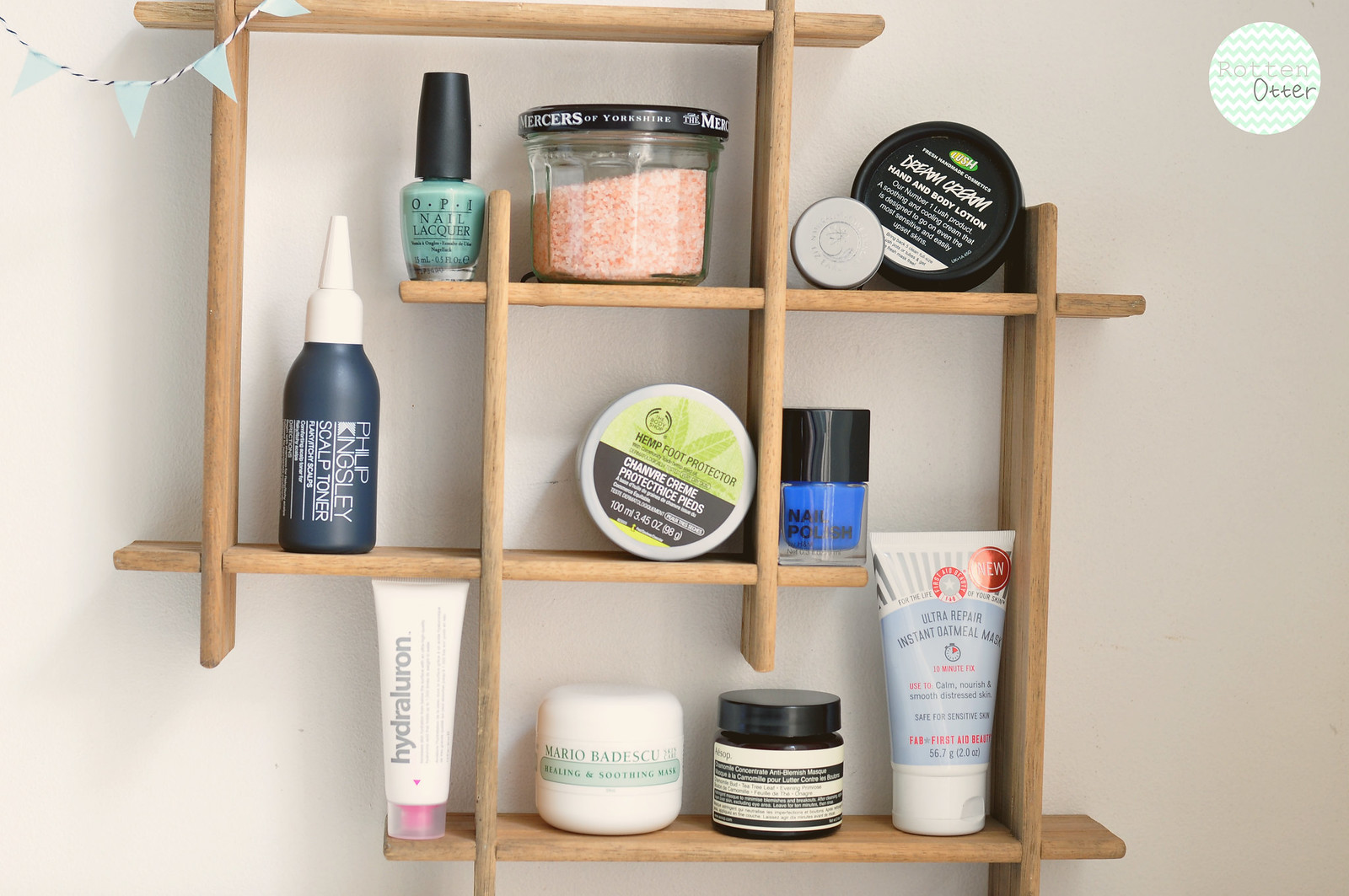This photograph captures a neatly arranged wooden shelving unit mounted on a light beige wall, showcasing an assortment of personal care products. In the upper right corner of the image, a logo featuring a mint green and white chevron pattern encircled by the words "Rotten Otter" — "Rotten" in a very light gray, and "Otter" in a dark gray, both in a handwriting-style font — adds a personalized touch to the scene. 

On the top shelf, a black jar of Lush's Dream Cream Hand and Body Lotion takes center stage. Next to it, a bottle of vibrant bright blue nail polish labeled simply as "Nail Polish" stands out without revealing its brand. Adjacent to the nail polish, The Body Shop's Hemp Foot Protector occupies a prominent position. 

Further down and to the right of the nail polish, a tube of Ultra Repair Instant Oatmeal Mask by First Aid Beauty is visibly positioned. Close by, a jar of Mario Badescu Healing and Soothing Mask is nestled, alongside a bottle of Philip Kingsley Scalp Toner, which is slightly overshadowed by the bottle of mint green OPI Nail Lacquer placed above it.

On the bottom left shelf, a tube labeled "Hydraluron" completes the well-curated collection. This detailed assortment of products highlights a well-thought-out approach to skincare and personal grooming.